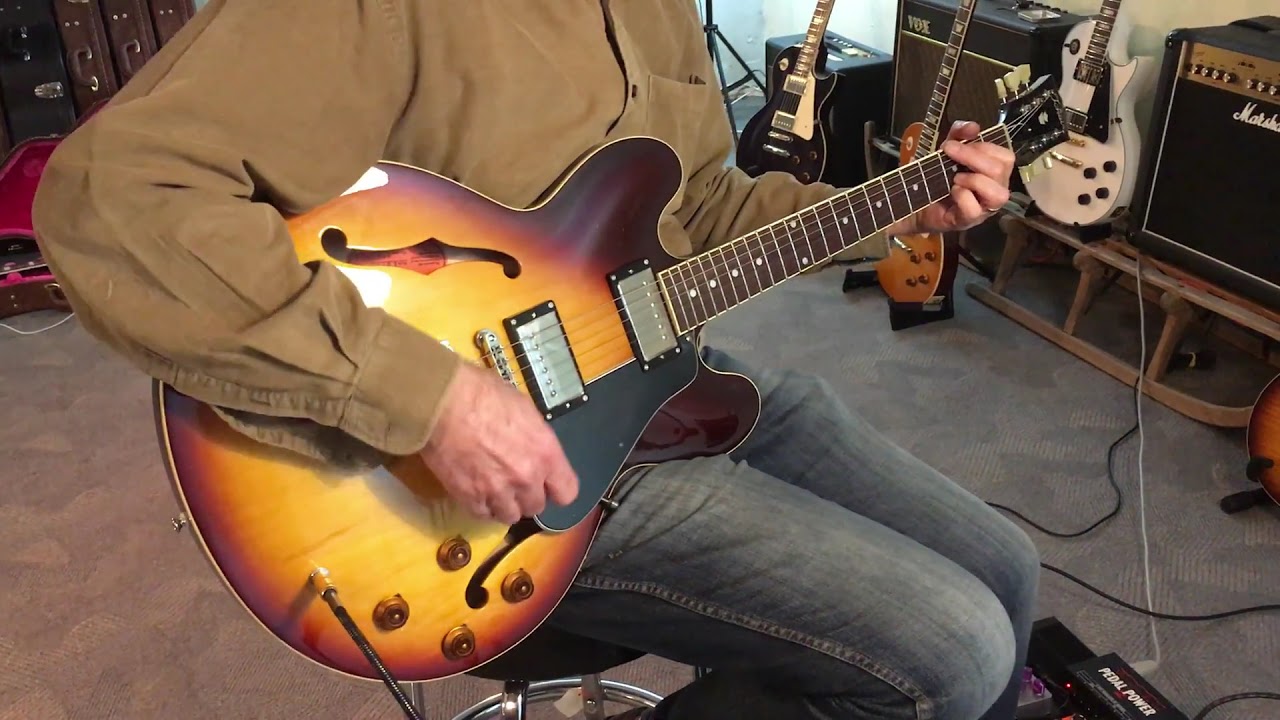This indoor image, likely taken in a personal music studio, features a man sitting on a stool, playing an enameled, shiny, yellow and reddish-colored guitar. The man, wearing a brown long-sleeve shirt with open cuff buttons and blue jeans, is centered in the image but only visible from the chest up and knees down. His right hand strums the strings while his left hand grips the guitar neck. The background reveals a carpeted floor and various musical equipment: two guitars on the ground and one on a stand to the right, accompanied by two speakers and a black equipment box. In the top left corner, additional carrying cases and gear are visible. Near the bottom right, a tangle of cords and a pedal labeled "Pedal Power" are in view, further emphasizing the studio setting. The overall color palette includes tan, brown, orange, yellow, black, white, blue, red, and silver.